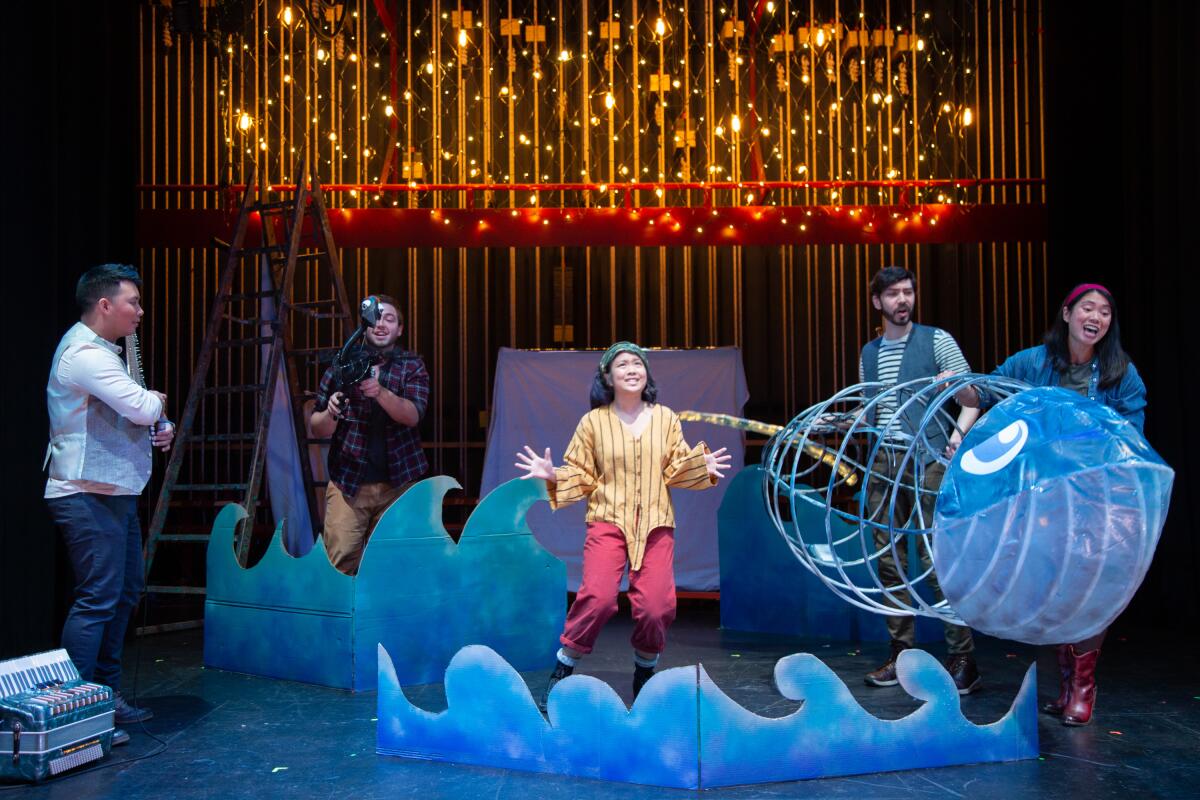The image captures a vibrant scene from a theatrical play, where five performers are actively engaging with the audience from the stage. At the center, a woman stands with her arms bent and palms facing the camera, conveying a sense of energy and action. She is dressed in eye-catching red pants and a yellow shirt, adding a burst of color to the scene. The stage setup includes a cardboard section at the bottom, creatively crafted to resemble water. On the right side of the stage, two individuals are seen holding a large, fish-shaped object, suggesting a thematic element related to the sea or fishing. Meanwhile, on the left side, a person stands in front of a ladder that is positioned toward the back of the stage. Behind this ladder, another performer holds an indistinct object, adding a layer of intrigue and complexity to the scene. The overall composition of the image depicts a dynamic and imaginative performance that captivates the audience's attention.